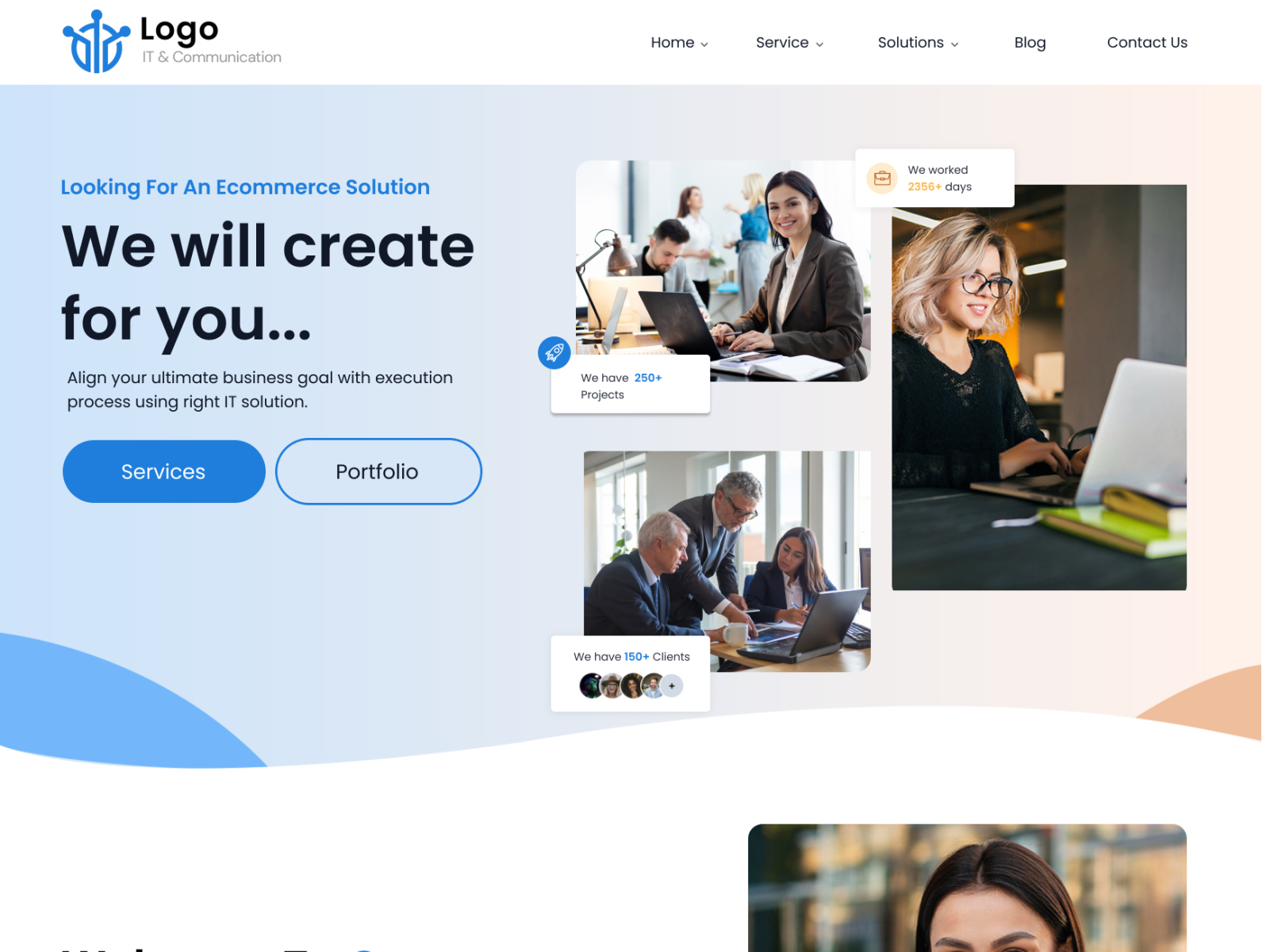The image features a slide or graphic design intended for an e-commerce solutions provider. In the top left corner, the text "logo" is displayed, accompanied by a minimalist logo of three lines with nodes at their ends. Beneath this logo, the text "IT and Communication" is prominent. The slide appears to be a homepage, with main navigation subsections including Home, Service, Solutions, Blog, and Contact Us. 

The layout is divided, with the left half predominantly in shades of blue and the right half in shades of orange and brown. Stock photos of people working in office environments are scattered throughout the design, with most of the subjects being young, happy women, engaged in computer-related tasks. Prominent call-to-action buttons labeled "Services" and "Portfolio" stand out, inviting user engagement. The overall theme suggests aligning business goals with the right IT solutions, aimed at enhancing execution processes for e-commerce.